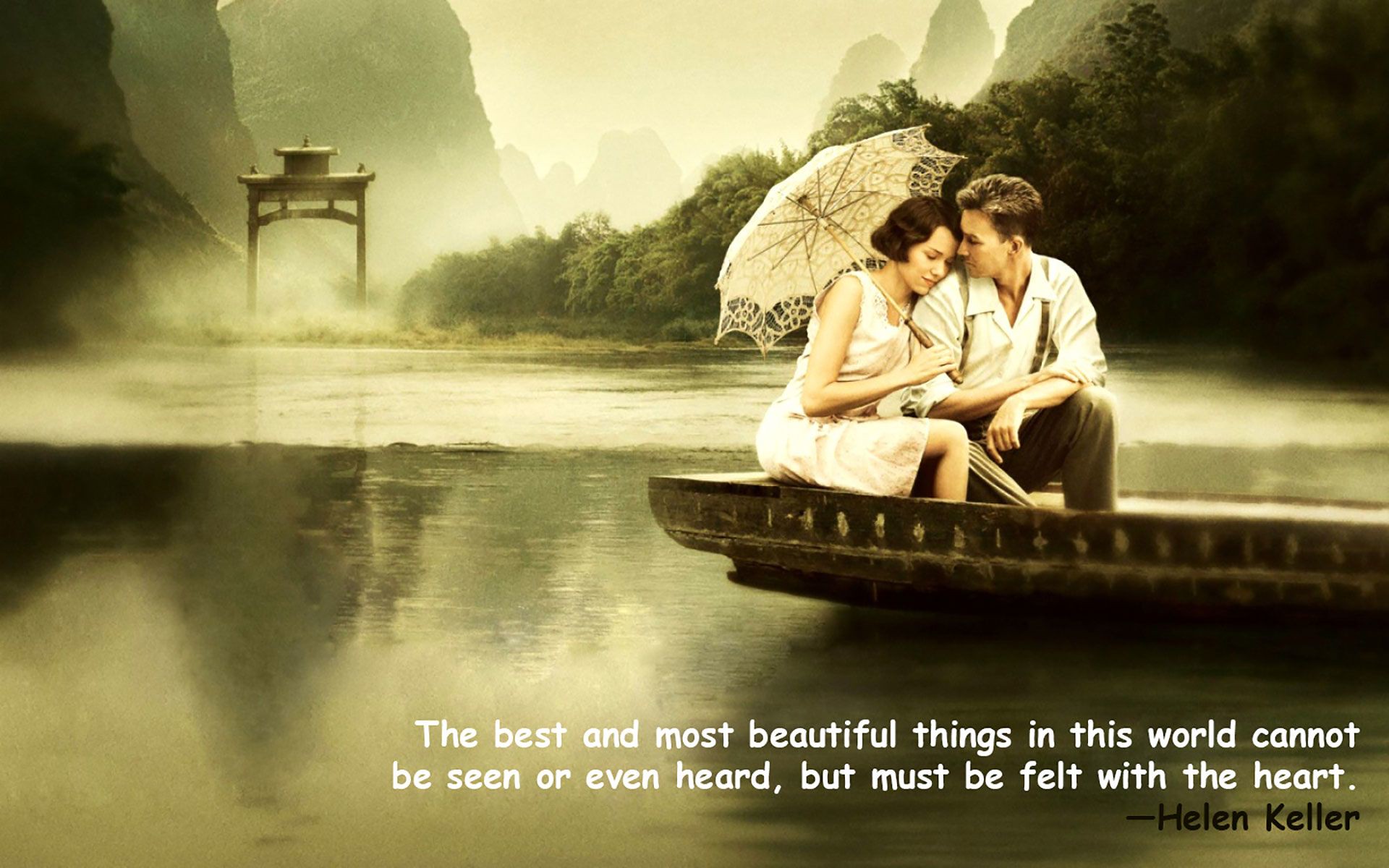In the image, a CGI-rendered young couple is seated on a boat drifting along a tranquil river. The river flows amidst lush greenery, mountain ranges, and misty hills. The woman, holding an umbrella, and the man, dressed in white with suspenders, share a tender moment. He presses his nose against her forehead while she looks down, conveying a sense of deep affection. The background features a mist-covered expanse with an Asian river setting, including a Chinese gate. The overall atmosphere is serene and somber, enhanced by the fog that envelops the scene. At the bottom of the image, a quote by Helen Keller reads: "The best and most beautiful things in this world cannot be seen or even heard but must be felt with the heart." The image combines elements of romance and tranquility, with a motivational message underlining its emotional depth. The colors are muted, consisting of black, brown, gray, tan, white, and olive tones, adding to the serene and poignant mood of the scene.